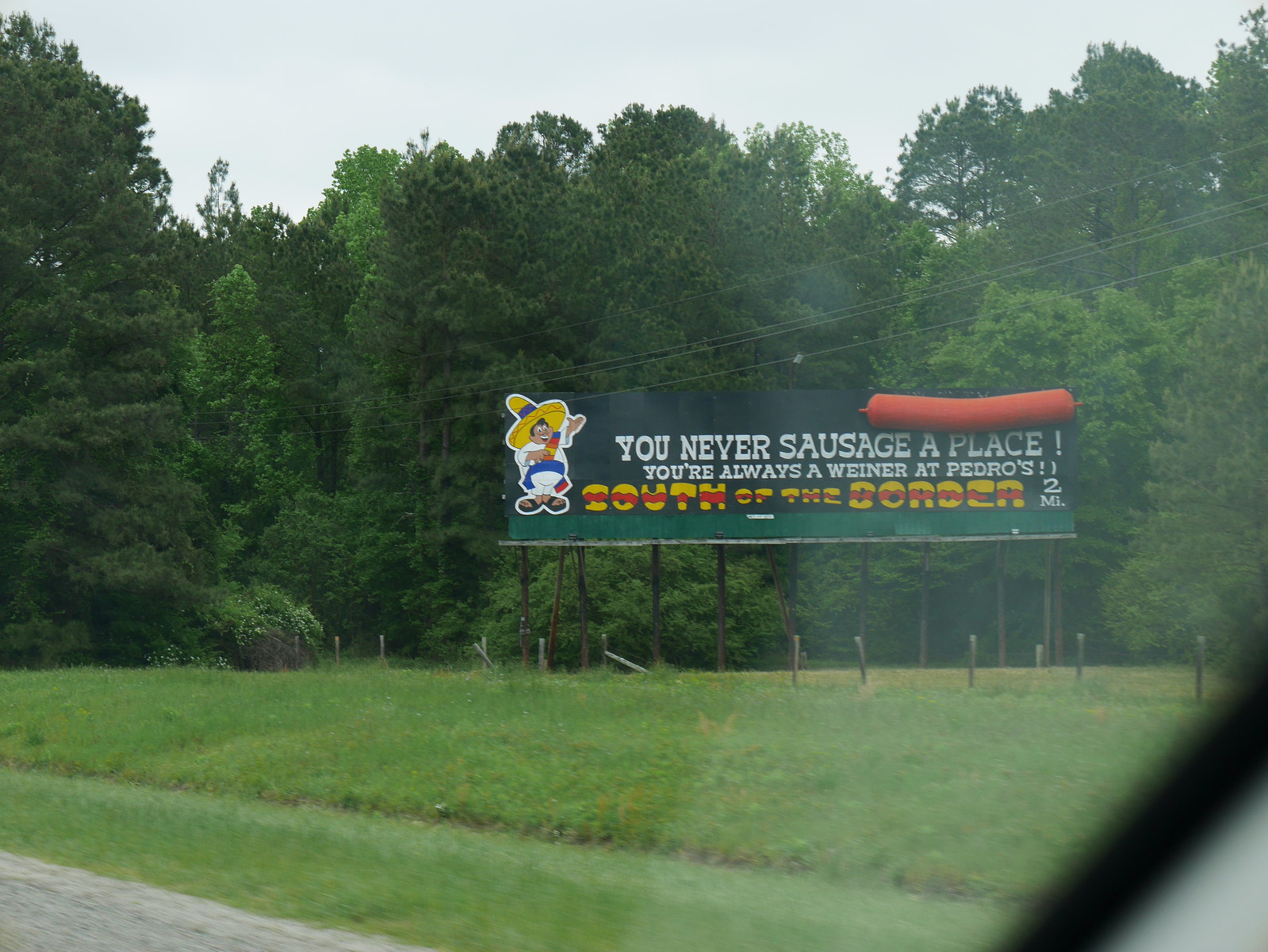The photo features an outdoor setting with a clear blue sky and a dense tree line of varying heights covered in green foliage. In front of the trees, there's a grassy area dotted with short poles and what appears to be a wooden fence with some wire. The focal point of the image is a large billboard supported by wooden posts. The top of the billboard is dark green, gradually lightening to a lighter green at the bottom. Prominently displayed on the billboard is the playful slogan, "You never sausage a place. You're always a wiener at Pedro's South of the Border," with "South of the Border" highlighted in yellow against a red stripe. Additionally, the message "two miles" is written in white. The billboard features a graphic of a reddish-brown sausage link at the top and a cartoon man dressed in a white outfit with black sandals, a blue sash over his left shoulder, and a sombrero, enhancing the vibrant and whimsical nature of the advertisement.